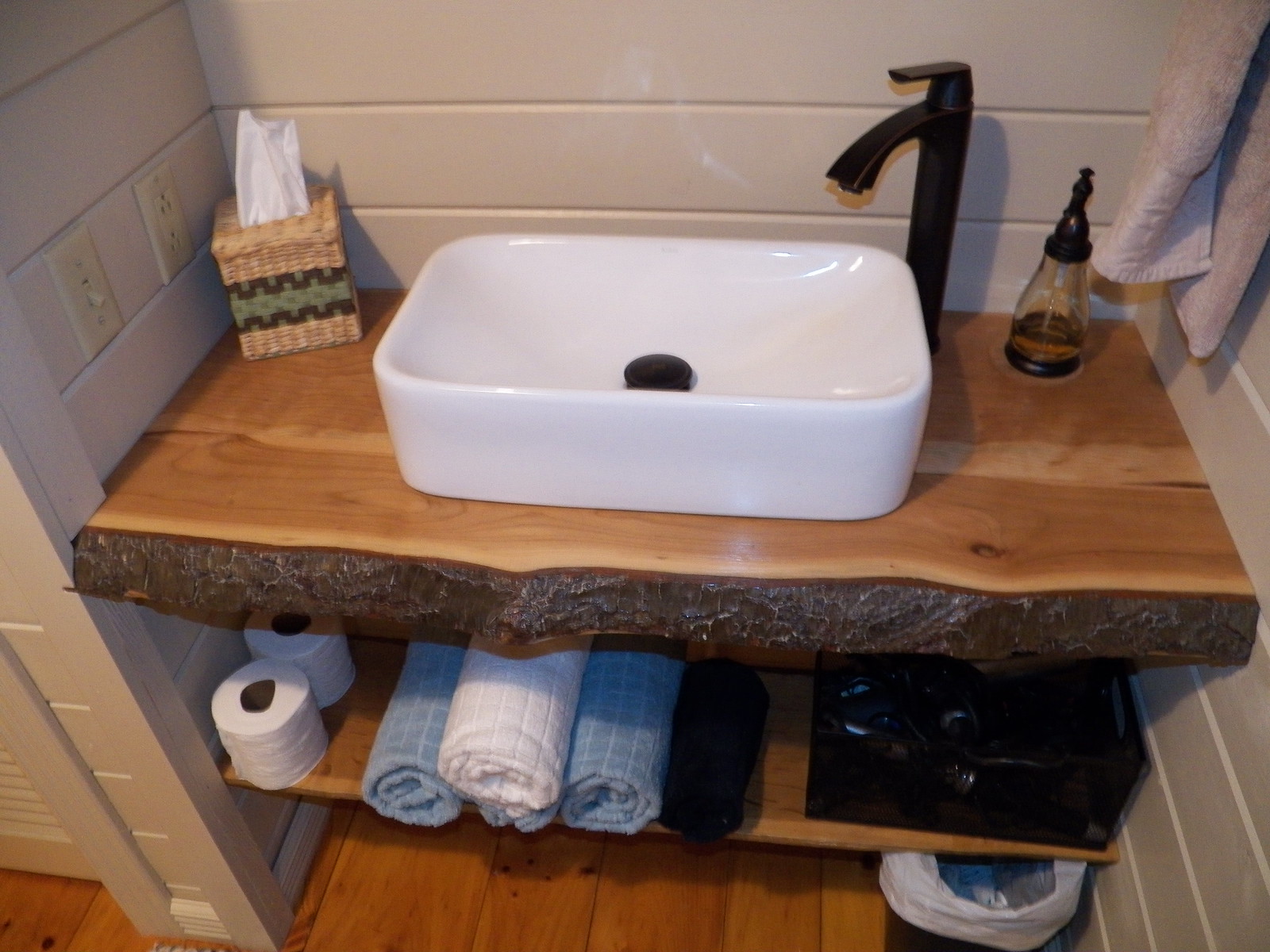This color photograph depicts a meticulously designed bathroom alcove. The rustic flooring features wide, finished pine planks adorned with natural knots, emphasizing an earthy aesthetic. The walls, crafted in a shiplap style painted white, offer a clean backdrop accentuating the overall calm ambiance of the room. 

Spanning the alcove is a robust, live-edge wooden countertop, approximately two inches thick. This medium-toned slab retains its natural bark edge, providing a raw, organic charm. Resting atop this natural masterpiece is a rectangular white porcelain vessel sink. Complementing the sink, in the back right corner, stands a tall, oil-rubbed bronze single-handle faucet, exuding a touch of vintage elegance.

Accenting the countertop are practical items including a pump soap dispenser and a tan woven tissue box cover, the latter housing a tissue peeking out from its cubical frame. An ivory-colored light switch and receptacle are mounted on the left wall, adding functional elements to the space.

The right wall features a hanging hand towel, neatly displayed for use. Below the countertop sits a slender shelf, which serves as additional storage. Here, neatly rolled towels in various hues of blue and white share space with a black mesh caddy, potentially holding a hair dryer. To the left of the shelf, a couple of extra rolls of toilet paper are neatly arrayed. Positioned under the right side of the shelf, a trash can with a white liner completes the scene, ensuring the alcove remains tidy and practical.